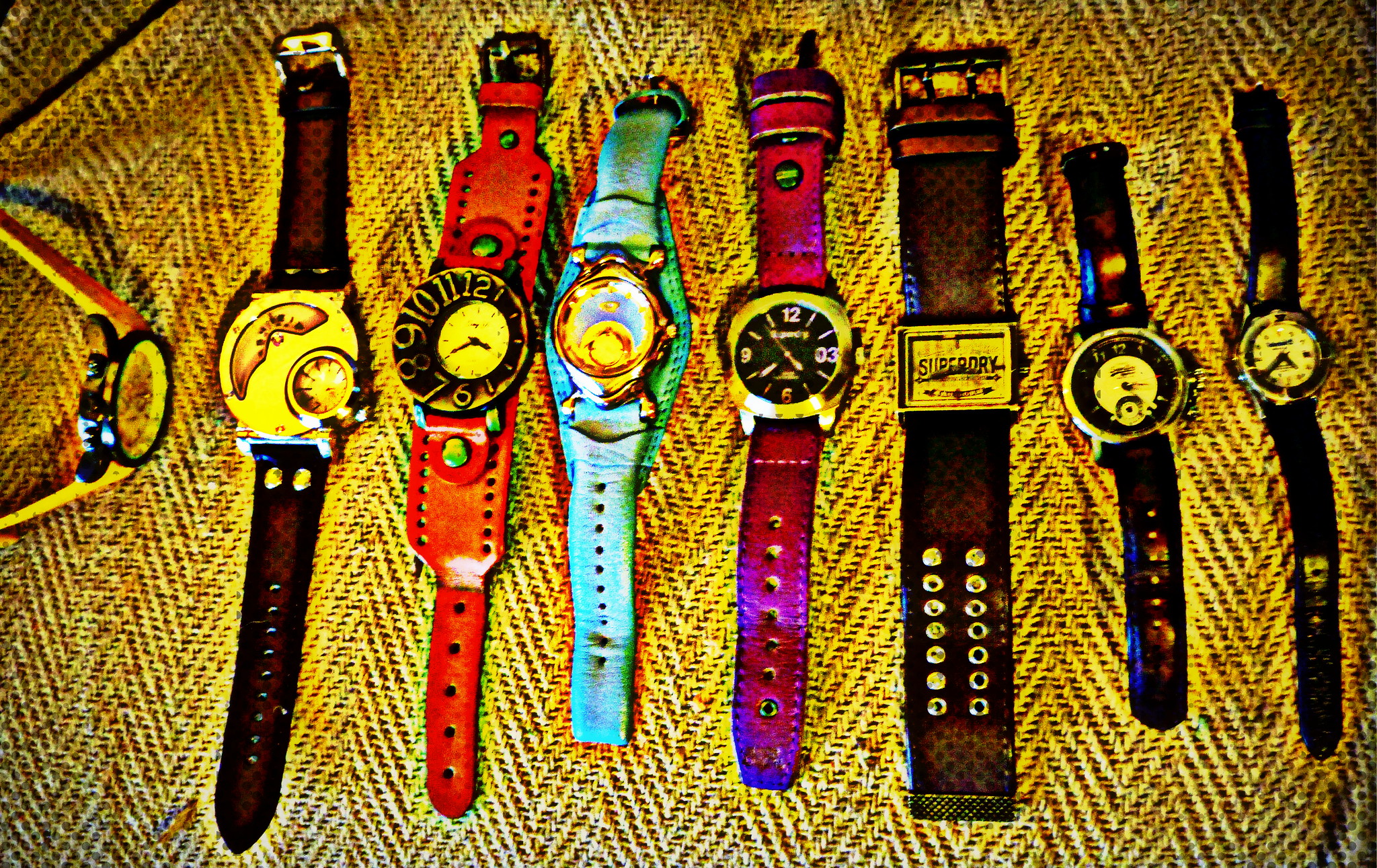This photograph depicts eight wristwatches meticulously arranged on a highly saturated yellow cloth with horizontal black stripes. The image, enhanced with a harsh contrast filter, distorts the colors, making them appear exceptionally bright and vivid. The watch on the far left is positioned on its side, displaying its brown leather band rather than its face and still partially buckled. The remaining seven watches are laid out flat with their faces up, showcasing a variety of designs and colors. 

From left to right, the watches feature different combinations: one with a brown leather strap and a yellow face, another red with a yellow face, a blue one with a yellow face, a reddish-brown watch displaying a black face, a brown watch with a square face, followed by two more brown watches. All watches have traditional clock hands rather than digital displays, and one prominently features the brand "Superdry." The photo's intense filter accentuates the colors, making the leather bands ranging in thickness, from medium to thick, stand out more starkly against the vivid backdrop.